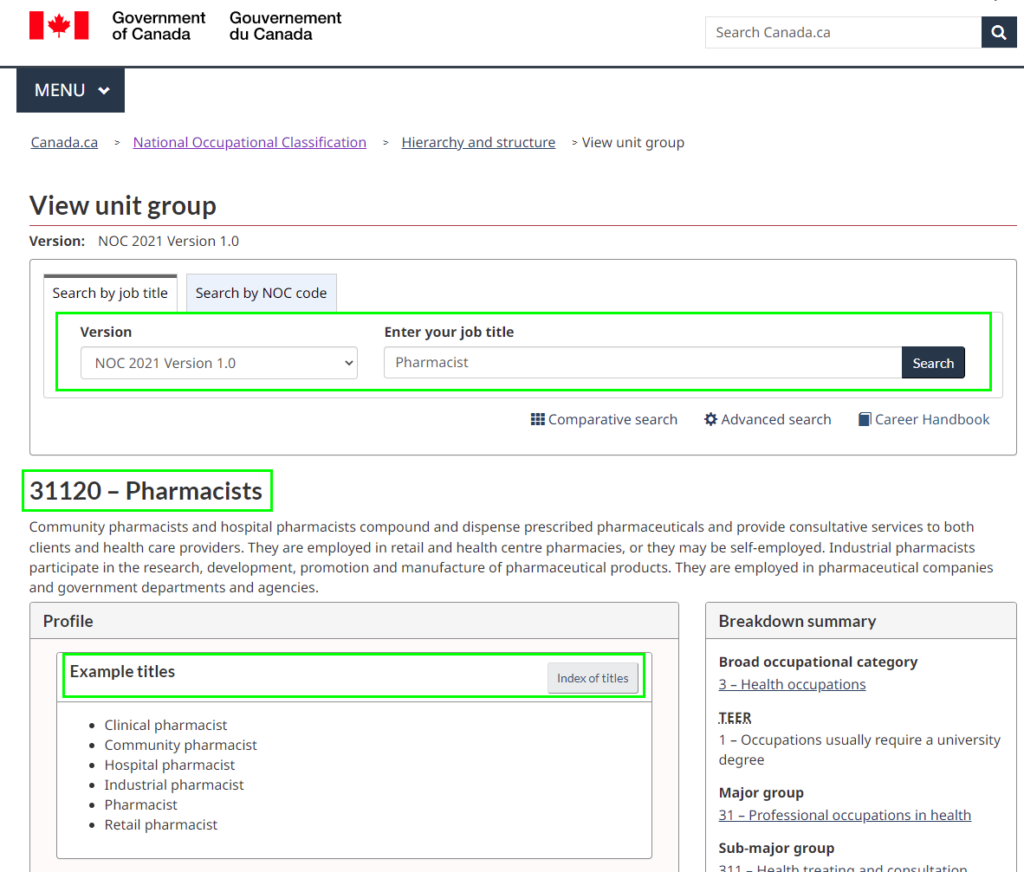In this image, we see a detailed view of the Government of Canada's website, specifically focused on the National Occupational Classification. The top right corner displays options for 'Search Canada.ca' and the main navigation menu. The webpage is titled 'National Occupational Classification,' highlighting the sections 'Hierarchy and Structure' and 'View Units Group' for the NOC 2021 version 1.0. 

Users have the option to 'Search by job title' or 'Search by NOC code.' In this instance, the job title 'pharmacist' has been entered, leading to a search for NOC code 31120. The page details roles such as community pharmacist and hospital pharmacist, describing their responsibilities in compounding and dispensing prescribed pharmaceuticals, as well as providing consultative services to clients and healthcare providers. These pharmacists are typically employed in retail and healthcare pharmacies or may be self-employed. 

Additionally, the page mentions industrial pharmacists, who are involved in the research, development, promotion, and manufacture of pharmaceutical products. They are employed by pharmaceutical companies, government departments, and agencies. The structured and comprehensive information aims to provide a clear understanding of the occupational roles and the contexts in which they operate.